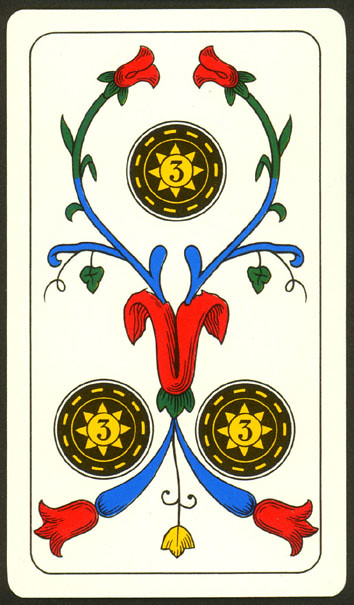The image captures the back of an ornate playing card, which is slightly longer than a typical deck card, hinting at its uniqueness. The card's design showcases three prominent black discs, each featuring a radiant gold sun at its center and encircled by a dotted gold line along the outer edge. Within these suns, the number "3" is clearly displayed, sparking curiosity about the card's significance—perhaps it belongs to a casino set or represents a "three of" suit in a custom deck.

Interwoven throughout the card are intricate vines that transition between blue and green hues. These vines sprout tulip-shaped flowers, with two positioned at the top and slightly larger ones at the bottom, adding a touch of elegance to the design. Dominating the middle section of the card is a draped red cloth, reminiscent of a sagging towel held by its ends, adding a striking contrast to the overall composition. Surrounding this central element are green leaves hanging from blue branches, interspersed with more pointed leaves from the green vines, completing the intricate and colorful botanical theme.